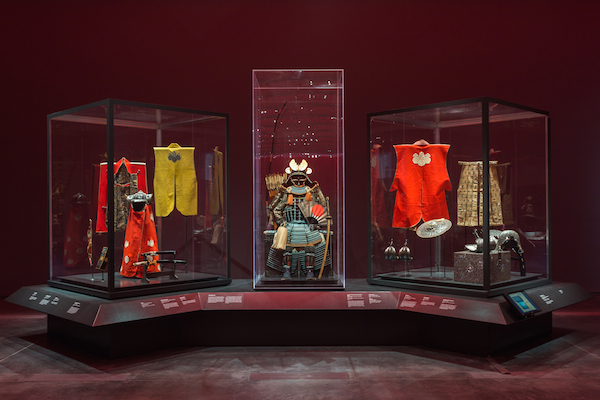This photograph captures a museum exhibit showcasing historical Japanese warrior attire and artifacts. Three transparent display cases sit prominently on a black podium atop a black floor, against a maroon backdrop. Each case displays different items and features little white labels in front of them. 

To the left, a nearly square black-framed case reveals various garments, including a striking yellow vest, red pants, and a matching red jacket. On the right, a similar black-framed case displays attire akin to the one on the left, featuring a red jacket and a beige vest.

The central case, rectangular and taller than the side cases, stands completely clear, containing an impressive samurai armor. The armor features a blue and dark brown statue of a seated warrior, equipped with a wooden sword to its left, a sheaf of arrows behind its right shoulder, a fan spread across its left thigh, and a white hat atop its head. The attention to detail and the carefully arranged items provide a compelling glimpse into the era's warrior culture.